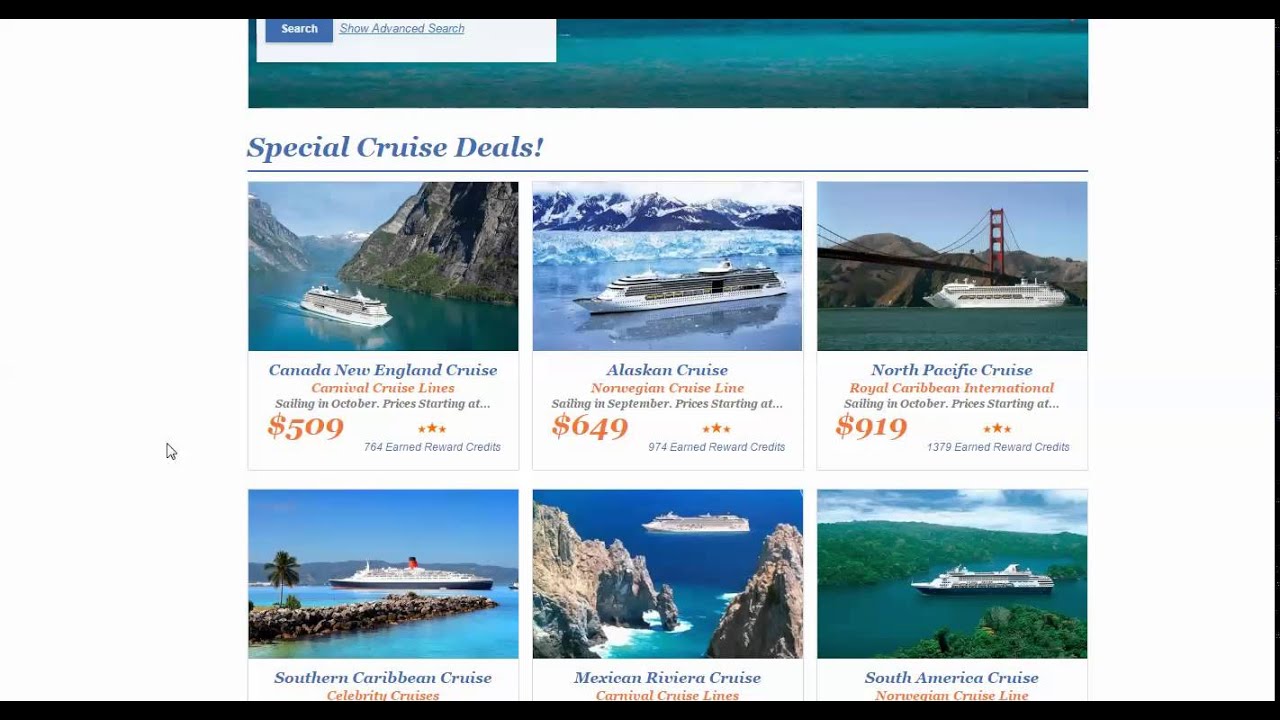This image showcases a webpage dedicated to travel, specifically highlighting special cruise deals. The webpage features a clean, white background adorned with numerous photographs of various cruise ships. At the top of the page, a teal blue banner is prominently displayed, containing a white search box and an option labeled "Show Advanced Search" for more detailed search criteria.

The centerpiece of the page is a bold, blue headline that reads "Special Cruise Deals!" Below this heading, several cruise options are listed, each accompanied by a photo of a ship set in its typical environment. The featured cruises include:

- Canada & New England Cruise for $509
- Alaskan Cruise for $649
- North Pacific Cruise for $919 (depicted with the iconic San Francisco bridge in the background)
- Additional cruises including a Southern Caribbean Cruise, Celebrity Cruise, Mexican Riviera Cruise, and Carnival Cruise Lines (partially cut off on the screen)

The last visible option is a South America Cruise with Norwegian Cruise Lines. Each cruise listing provides a small, picturesque screenshot portraying the cruise ship against a backdrop relevant to its itinerary, such as majestic mountains, serene oceans, or lush forests.

Overall, the webpage evidently offers a wide variety of cruises from different cruise lines, catering to various destinations and price points.